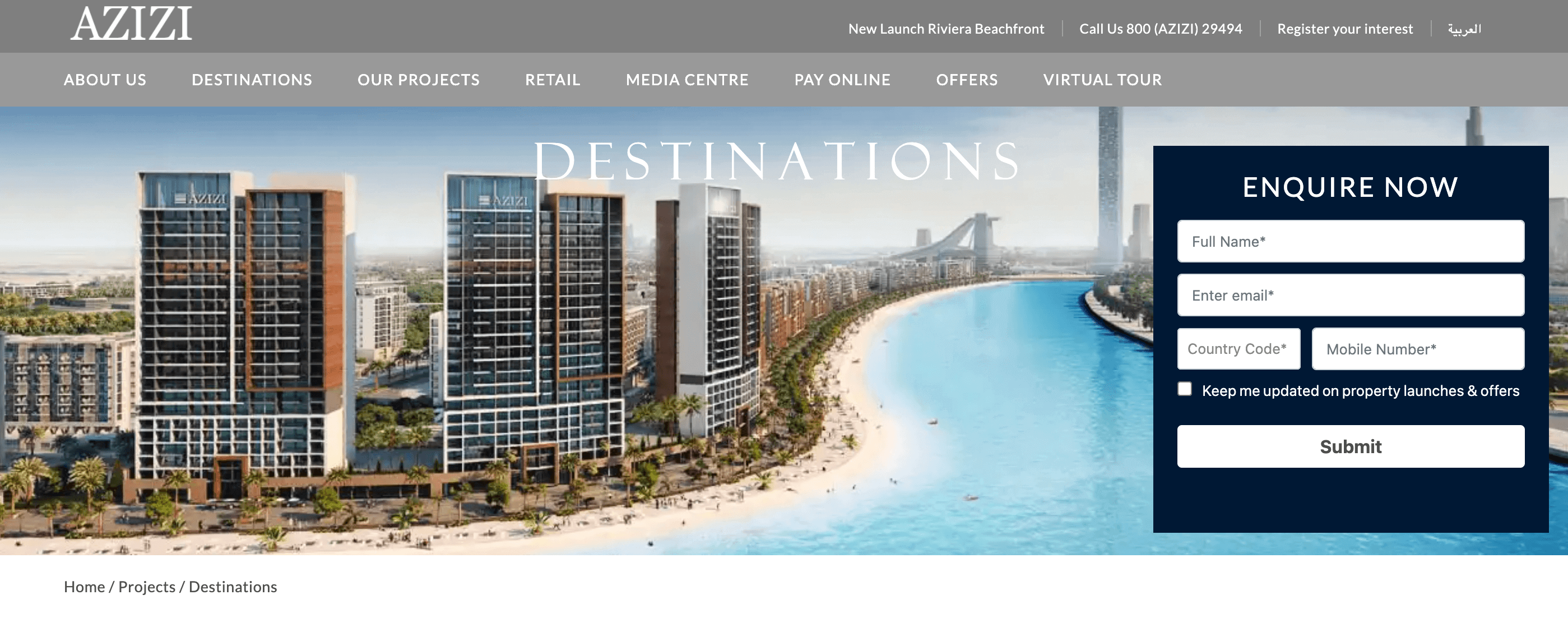The image on the Azizi website prominently features a stunning, expansive view of a picturesque waterfront scene. The vibrant, crystal blue water captures immediate attention, providing a refreshing contrast against the surrounding landscape. To the left, a sandy beach gently slopes into the water, creating a natural gradient that invites viewers to imagine the tactile sensation of sand beneath their feet. Towering buildings, possibly apartments or business complexes, rise up behind this sandy stretch, framing the scene with an urban touch.

The embankment gracefully curves around the waterway, leading the eye toward the background where a couple of tall towers punctuate the skyline, their industrial appearance reminiscent of smokestacks. On the right bank, a well-maintained concrete sidewalk suggests a promenade, perfect for strolling along the water's edge.

Overlaying this serene vista, Azizi's website interface features a promotional highlight titled "New Launch Riviera Beachfront," along with navigation options including "About Us," "Destinations," "Products," "Retail," "Media Center," "Pay Online," "Offers," and a "Virtual Tour." This multifaceted layout not only showcases the beauty of the waterfront but also provides users with comprehensive information and services.